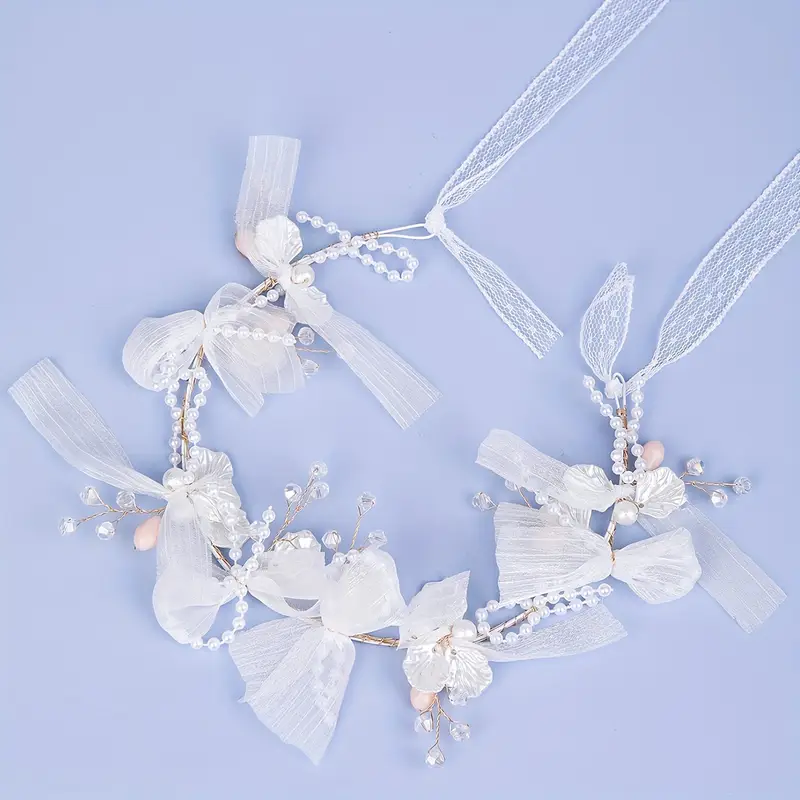The image features a delicate headpiece, likely a bridal or special occasion hair ornament, set against a periwinkle blue background. The ornament, resembling a tiara or headband, has an open, round shape with textured white gauzy ribbons tied around it. These ribbons extend to hang down over the chest when worn. Adorned with strings of crystal beads and glass sequins, this headpiece also includes clear beads on stems that give the appearance of tiny flowers. The base appears to be silver, adding an elegant foundation to the intricate beaded work and ribbon decorations. At the ends, there are loops with more white ribbons, some of which are lacy and shimmering, creating a sophisticated and detailed design.